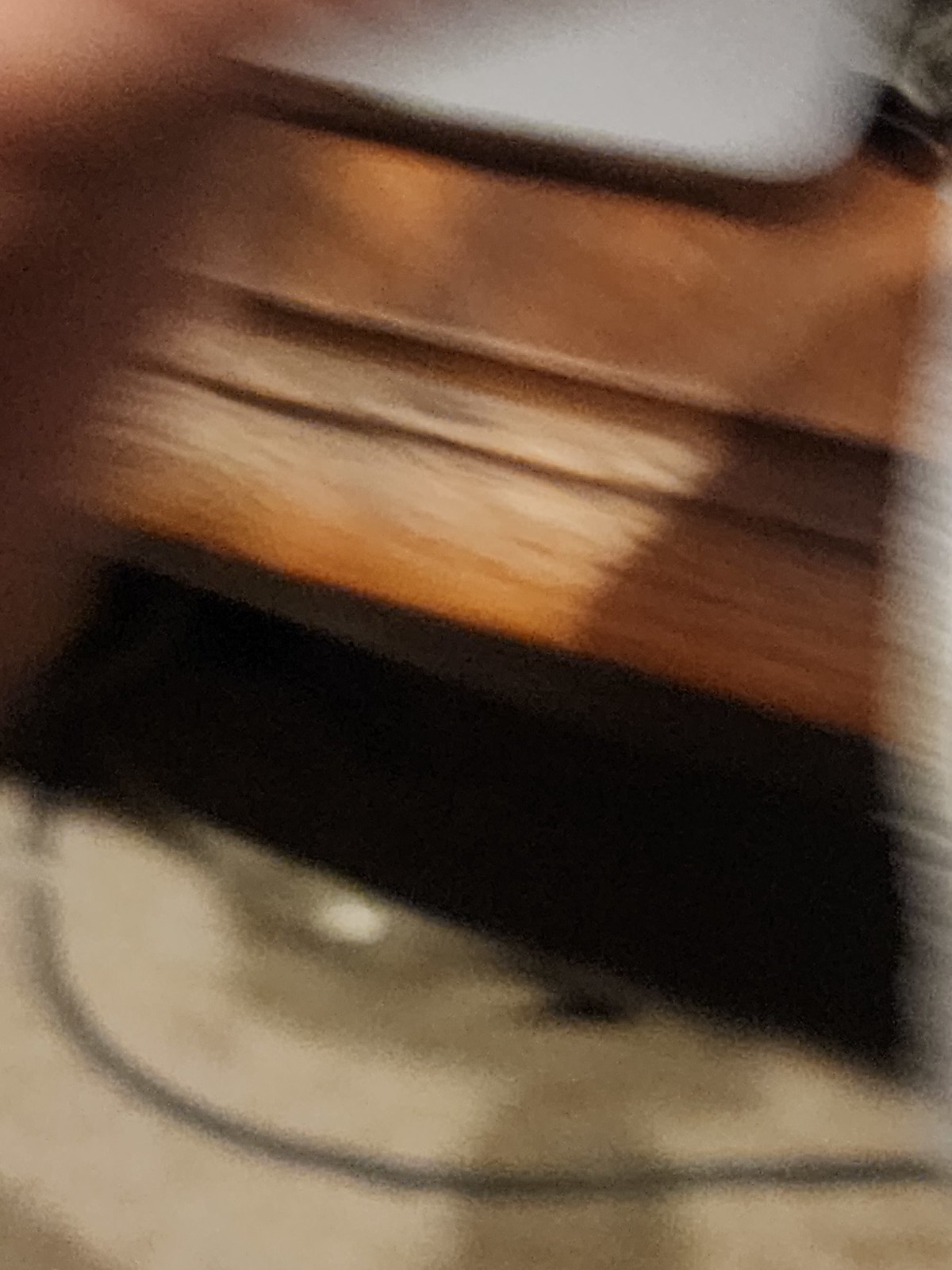The photograph is quite blurry and grainy, with heavy shadowing present throughout. At the bottom, there is a white object with a black line running through its middle. Above that lies a solid black layer, which is followed by another black line and then a section featuring light caramel and white-tan coloration. Higher up, there is a coffee-colored brown area with caramel-like swirls. Above this, a squared-off, gray object can be seen. In one part of the image, a portion of a person's hand is partially visible, showing a flesh-toned color. Due to the poor quality of the image, it is difficult to determine what the object might be, though it could possibly be a wallet.